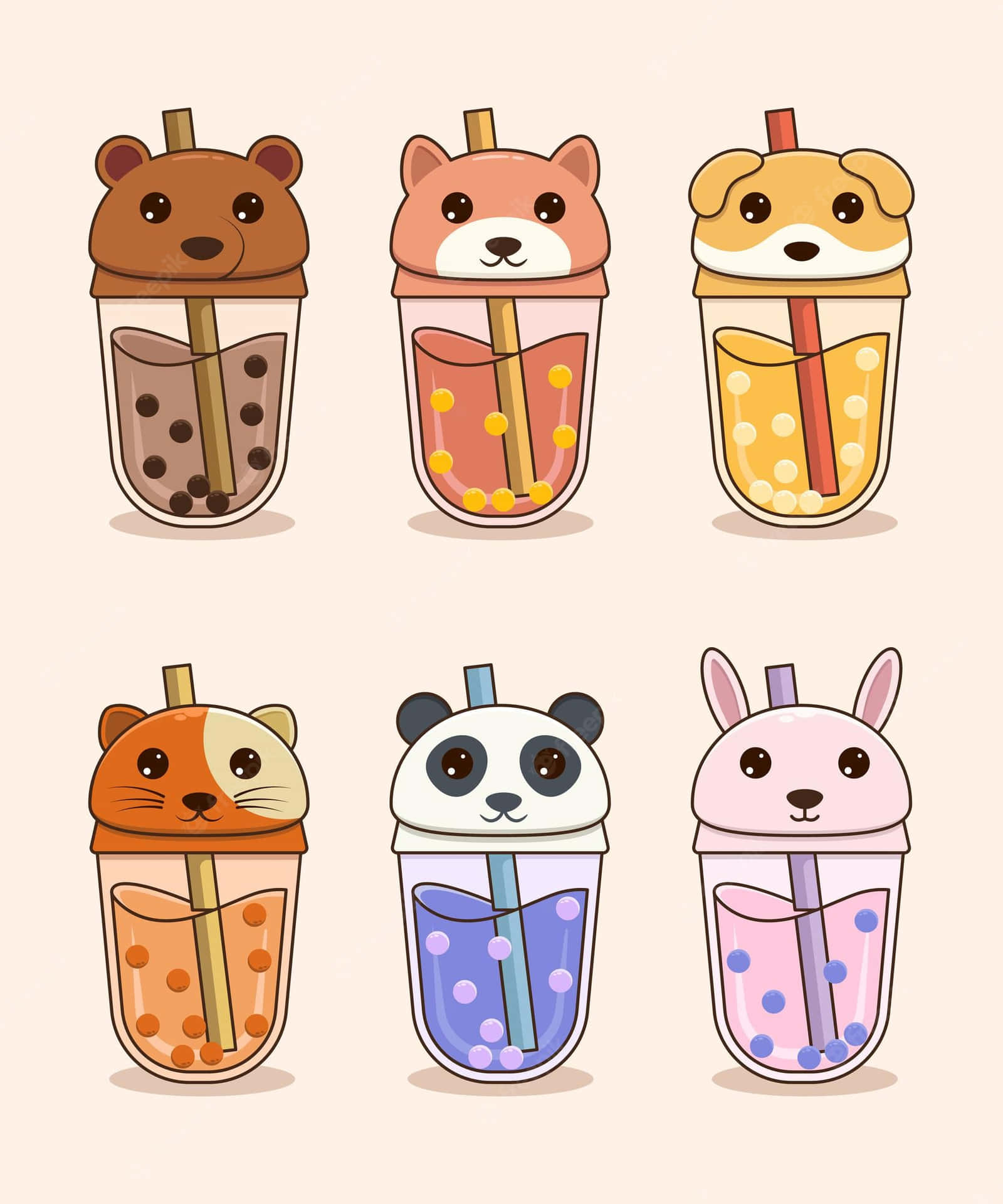The image depicts six whimsical, animated-styled boba cups against a beige background, each featuring a different animal character and uniquely colored boba tea. At the top left is a dark brown boba cup with a grizzly bear face, filled with medium-brown liquid and topped with a brown straw. To its right, in the middle, is a shiba inu themed cup filled with yellow liquid and white boba pearls, paired with an orange straw. At the top right, there is a beagle cup that also holds yellow liquid with lighter yellow spots and has an orange straw.

On the bottom left, there is an orange and white cat cup, featuring light orange liquid with darker orange boba pearls and a beige straw. In the middle of the bottom row, a panda cup contains light purple liquid with darker purple boba beads, and a blue straw. Finally, at the bottom right, a bunny cup is filled with pink liquid and purple boba dots, completed with a purple straw. All cups and their vibrant liquids create a charming and colorful display of animated boba beverages.